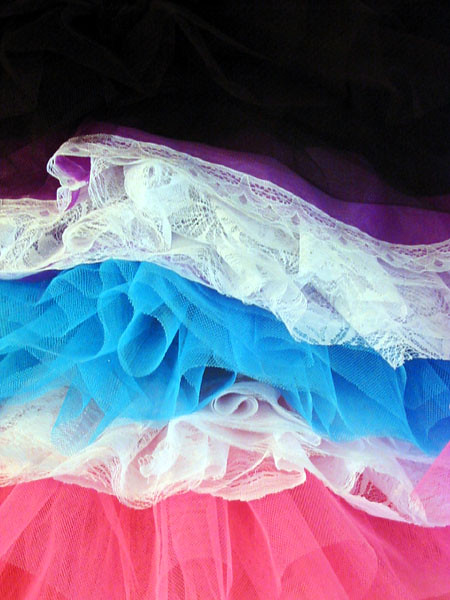The image depicts a stack of intricately layered fabrics, each folded and ruffled, showcasing a progression of colors and textures from bottom to top. The bottommost fabric is a pink tulle, followed by a white lace fabric. Above these, there is a blue tulle fabric, and then a distinct two-layered fabric with sheer white at the core, encased in purple fabric. Topping the stack is a black sheer tulle fabric. The fabrics appear meticulously stitched, new, and unused, with the ruffles adding a touch of elegance. The background of the image is completely dark, emphasizing the vibrant and delicate fabrics that dominate the view, giving the impression of a well-composed and possibly artistic photograph or painting.